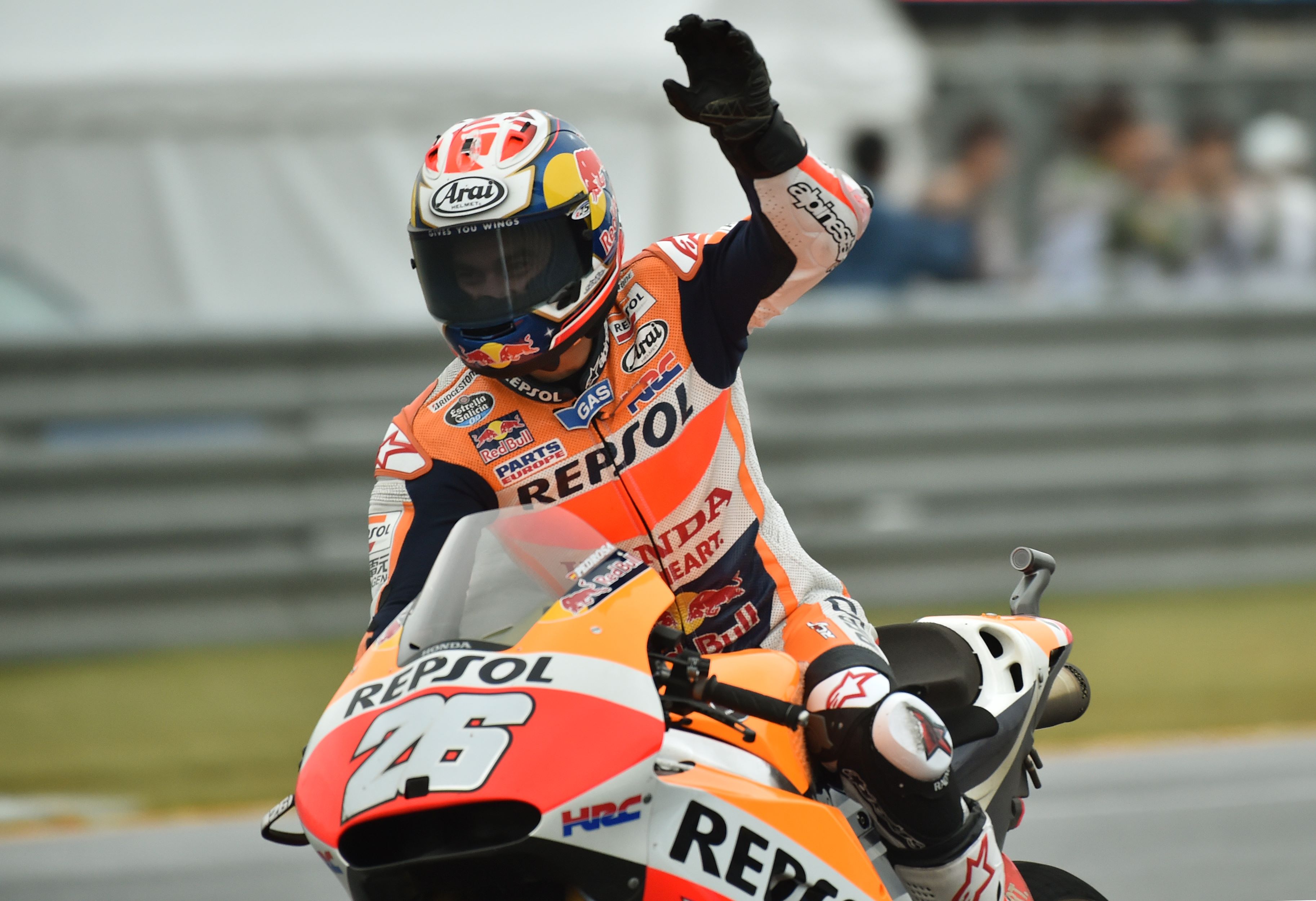In this image, we see a professional motorcyclist captured in a dynamic moment during a race. The rider is prominently wearing a brightly colored racing suit in shades of red-orange, orange, white, and black, adorned with numerous sponsor logos including Repsol, Honda, Red Bull, Arai, and Parts Europe. The suit prominently features "Repsol" in black and "Honda" in red lettering. The motorcyclist also dons a matching helmet with a dark visor and "Arai" emblazoned on the front.

The racer is seen leaning forward on the motorcycle while raising his left arm, possibly in a wave, showcasing black gloves on both hands. The motorcycle itself mirrors the color scheme of the suit with a combination of orange, red-orange, white, and black. The front cowling of the bike displays a clear windshield and a bold number "26" in white against an orange-red background.

The scene is set on a gray paved track, framed by a green strip and a corrugated metal fence in the background, which is slightly out of focus. Beyond the fence, one can discern a white tent and some indistinct spectators, adding to the lively atmosphere of the racing event. Despite the motion, the clarity of the image is high, with vibrant colors and ample lighting emphasizing the detailed visual elements.